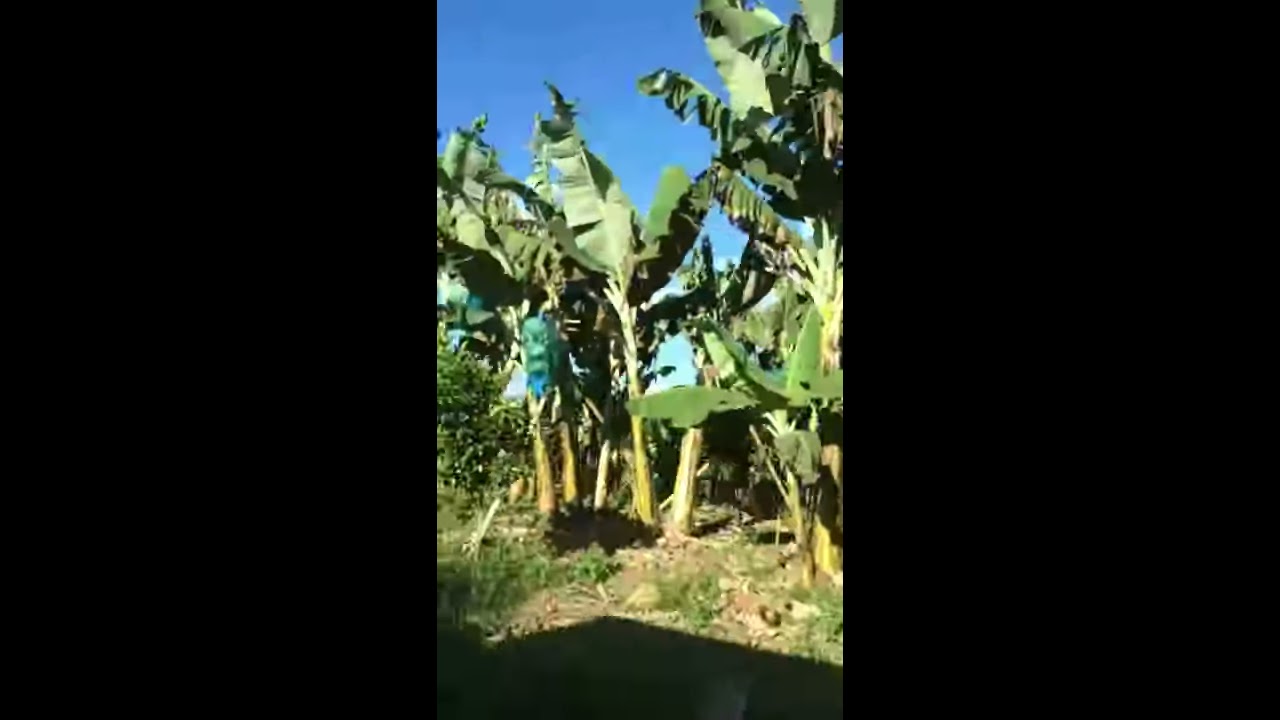A vibrant and sunny outdoor scene showcases a group of 6 to 8 banana trees with large, lush leaves at their tops. Set against a completely clear, blue sky, these trees rise from a dirt area interspersed with patches of green grass and weeds. The shadows cast by the sun attest to the bright, cloudless day. To the left side of the image, a small tree can be seen. Wind gently rustles the banana tree leaves, which appear to be partially protected by green and blue fabric. In the background, additional shrubs add to the rich, green landscape. The image is characterized by its striking contrasts between the vivid greenery of the plants and the deep blue of the sky, giving a fresh and lively feel to the photograph.